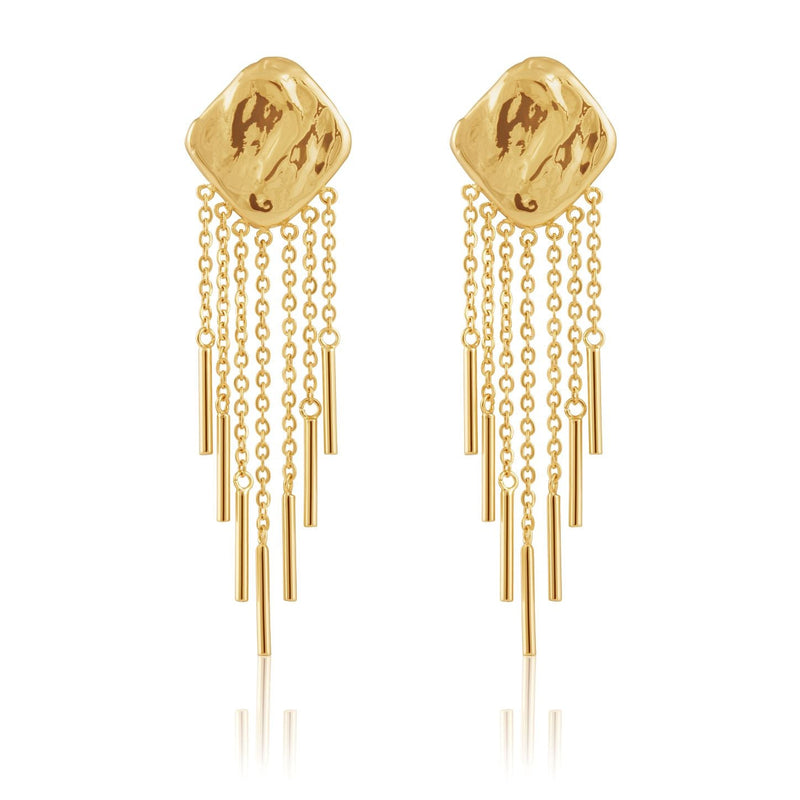This close-up photograph depicts a pair of gleaming gold earrings set against a stark white background, their reflections subtly visible below. Each earring features a diagonal, diamond-shaped top, embellished with a smooth, slightly textured finish and light brown speckles. From the base of this diamond, seven delicate gold chain links gracefully dangle, each linked to a small, tubular gold piece. These tubes are arranged to form a descending gradient from the outer edges inward, creating a visually appealing staggered effect. The overall design, intricate and sophisticated, suggests the earrings may be showcased in an advertisement, highlighting their luxurious and reflective qualities.